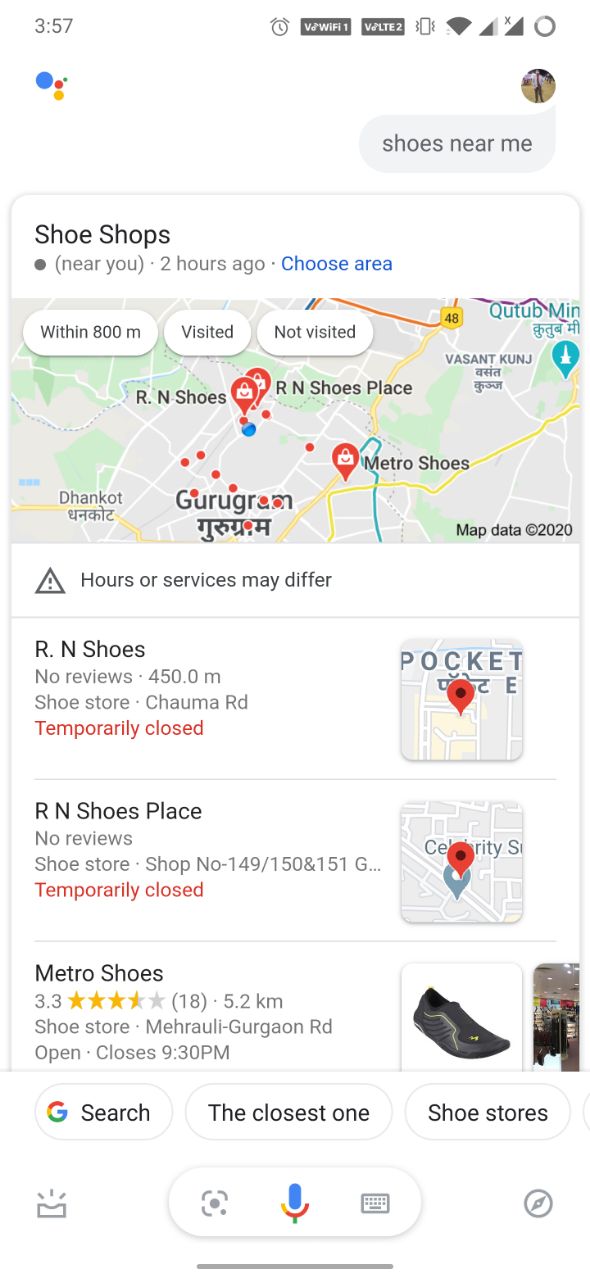This screenshot captures a mobile device displaying a navigation app in use. The user has entered "shoe shops" as their search criteria. The app is showing three shoe shops available nearby. These shops are named "Orange Shoes," "Orange Shoes Place," and "Metro Shoes," all located within close proximity to each other. The screenshot indicates that the location is likely outside the United States, although the exact city is not specified. The map at the top of the page prominently highlights the positions of these three shops.